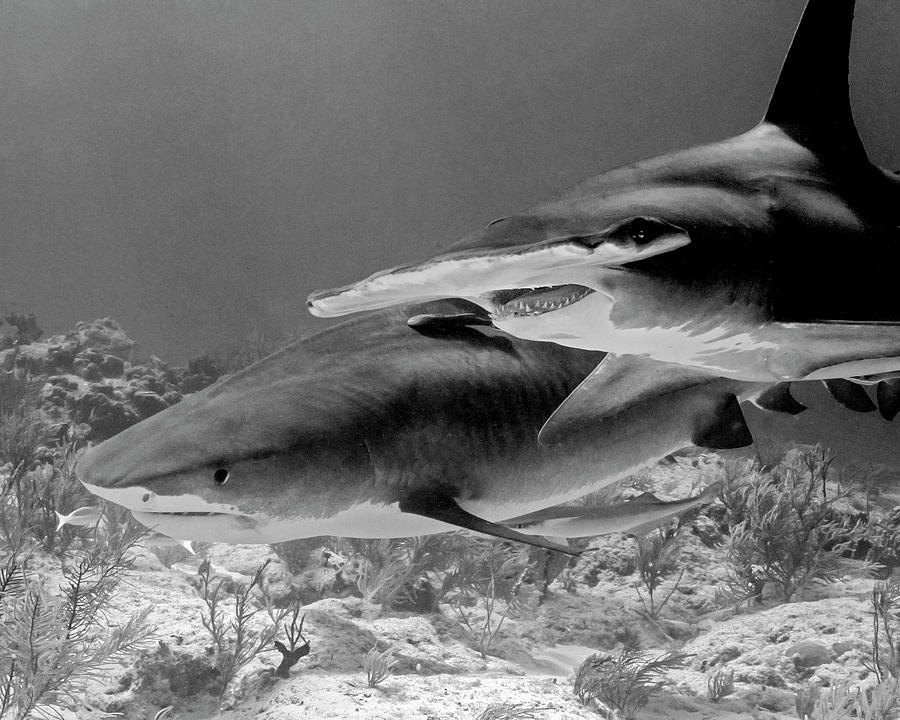This grayscale underwater photograph vividly captures two sharks prowling near the ocean floor, surrounded by an array of marine flora and rocky terrain interspersed with sandy patches. In the background, partially obscured by a coral reef, swims a typical great white shark with its distinctive black dorsal side and white underbelly. The great white's mouth is slightly open, revealing razor-sharp teeth, and a small pilot fish can be seen hovering just beneath it. Closer to the forefront is a formidable hammerhead shark, easily identifiable by its elongated, pointed snout and prominent vertical dorsal fin. Its mouth is agape, displaying several rows of sharp teeth and a striking black beady eye. Both sharks are oriented in the same direction, gliding stealthily through the underwater landscape, amidst the various rocks, ocean plants, and occasional small fish that populate the serene but haunting seafloor.